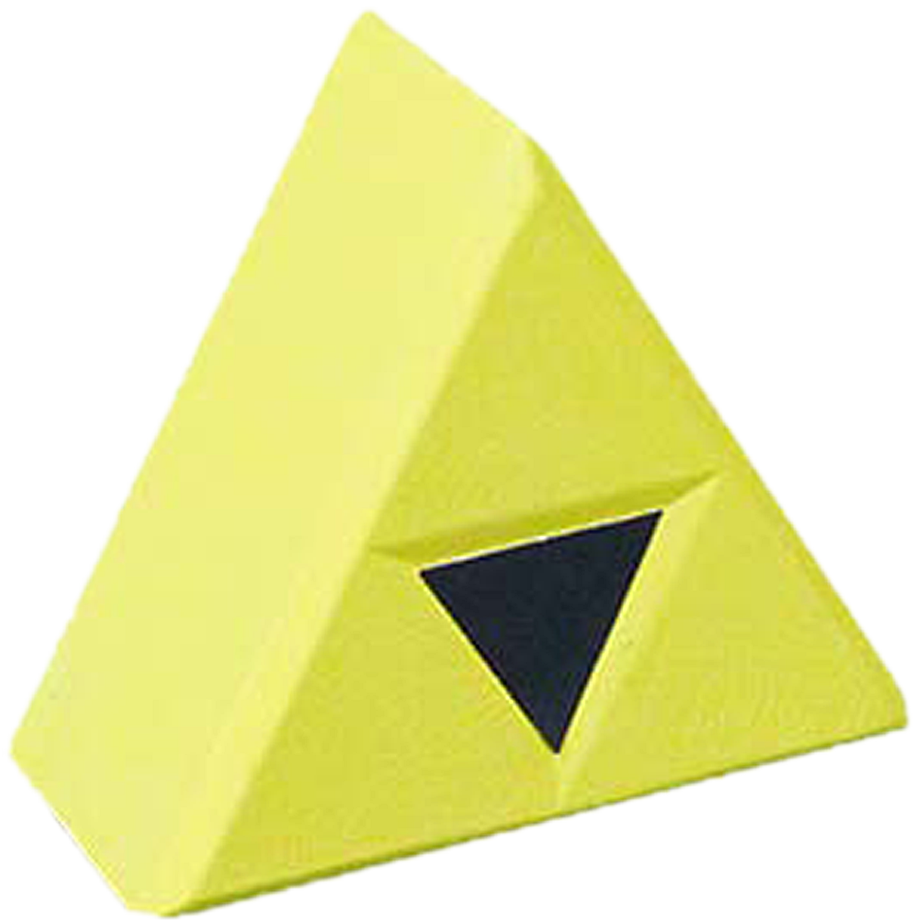The image displays a three-dimensional representation of the Triforce from the video game *The Legend of Zelda*. Positioned against a white background, the golden yellow triangular object stands upright with its apex pointing upwards and its base resting solidly at the bottom. The side facing directly towards the viewer is a slightly darker shade of yellow, almost verging on green, while the other visible face is lighter in hue. 

On the front face of this three-dimensional triangle, the iconic Triforce symbol is clearly displayed. This symbol comprises three smaller golden yellow triangles arranged such that an upright triangle sits in the center, flanked by two other triangles positioned on its left and right ends, also pointing upwards. Within the negative space created by these three triangles, another smaller black triangle is oriented upside down, with its point directed downwards. The overall structure rather resembles a wedge of cheese sold in stores, notable for its sleek, unadorned sides and distinctive, centrally-placed symbol on the front.